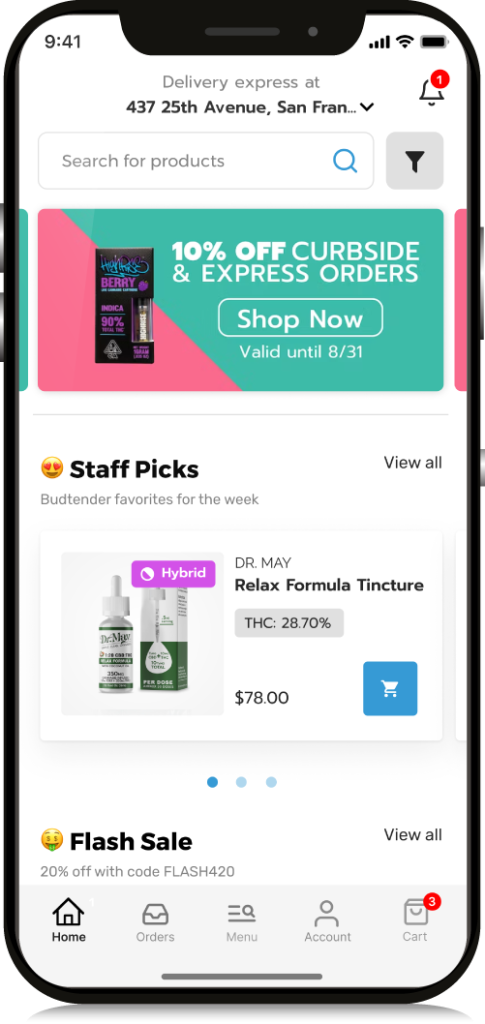**Caption for Screenshot of Mobile App Interface:**

The screenshot captures a mobile app interface of a delivery service, displayed on a smartphone. The phone shows the current time as 9:41, with full signal strength and battery. Prominently, the top of the screen indicates the current delivery hub as "Delivery Express at 437 25th Avenue, San Francisco," suggesting this is where the orders are dispatched from.

A vibrant teal and pink banner spans across the screen, announcing a "10% off curbside and express orders" promotion valid through August 31st. Adjoining the banner is an image hinting at package deliveries, with an adjacent similar banner partially visible, indicating more promotional content accessible by scrolling horizontally.

Above the promotional banner, a search bar invites users to browse for products, flanked by an unidentifiable button. Just beneath the banners, a section titled "Staff Picks" showcases "Budtender Favorites for the Week," featuring a product named "Relaxed Formula Tentacure" priced at $78.99, which can be swiftly added to the cart. Following this, a highlight on flash sales for additional items suggests a dynamic, potentially pharmacy-related service.

This detailed layout hints at a user-friendly shopping experience tailored for quick and efficient product selection, alongside enticing deals and staff recommendations.